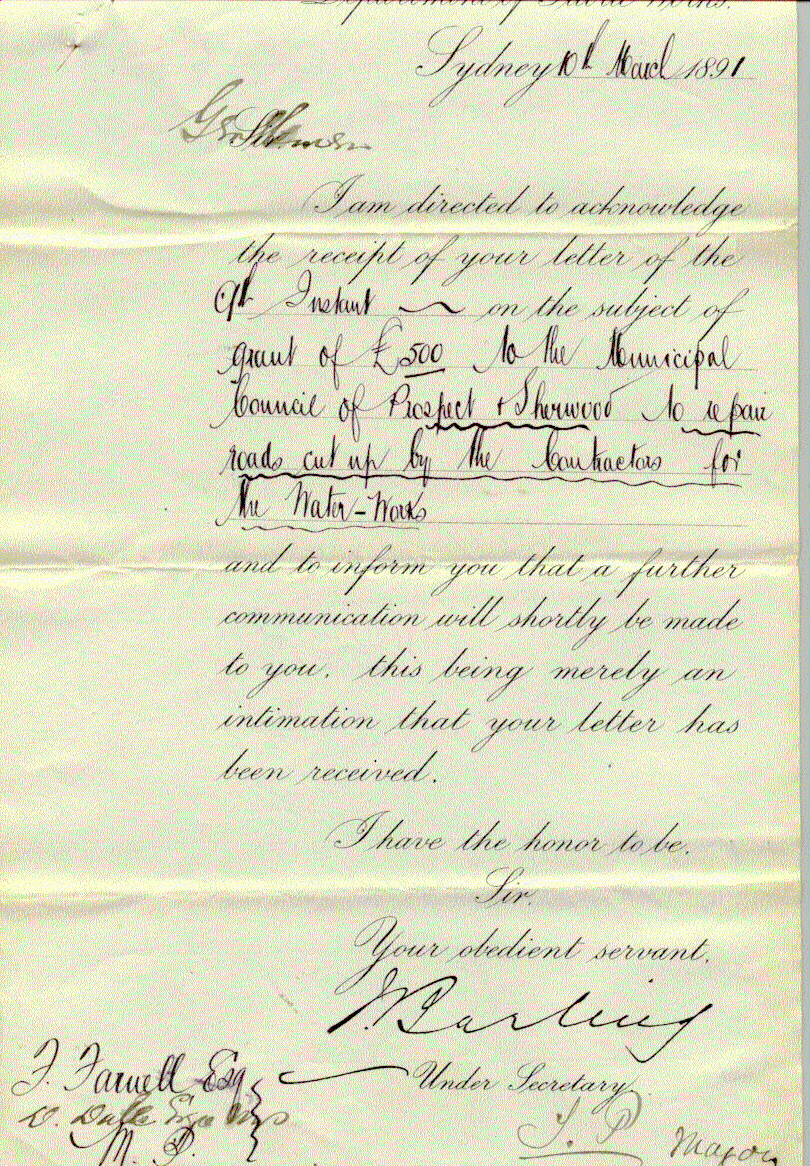The image depicts an old, off-white sheet of paper with cursive handwriting in black ink, dating back to 10th March 1891. The letter, dated in Sydney, Australia, acknowledges the receipt of a previous correspondence concerning a grant of 500 pounds to the Municipal Council of Prospect in Sherwood. Despite the text being somewhat difficult to read due to the age and cursive style, parts of the letter are clear: "I am directed to acknowledge the receipt of your letter... on the subject of grants of 500 pounds to the Municipal Council of Prospect, Sherwood... and to inform you that a further communication will shortly be made to you. This being merely an intimation that your letter has been received. I have the honor to be your obedient servant." The document is signed at the bottom by a secretary or a similar official. The paper shows signs of aging, including yellowing and slight compression, which adds to its vintage appearance.